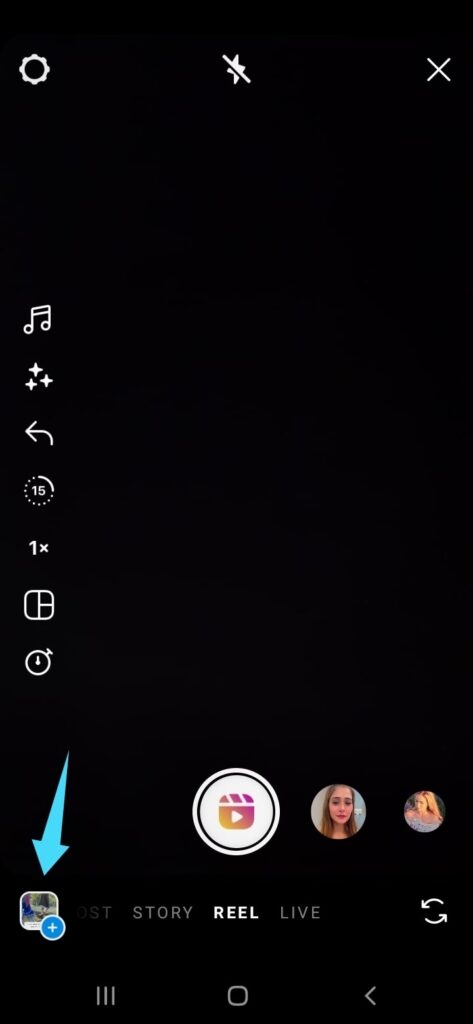This image is a vertical screenshot of what appears to be a cell phone screen with a solid black background and white text. In the upper left corner, there is a circular icon, and to its right is an icon that likely indicates 'no flash,' represented by a lightning bolt with a diagonal line through it. An 'X' is situated in the upper right corner of the screen.

At the bottom of the screenshot, there is a small square featuring an unclear photo with a large blue arrow pointing downward above it. Next to the square is a blue circle containing a plus sign.

To the right of this blue circle, there is a white icon that looks like a play button. Further to the right are images of two women: one with long brown hair and the other with long blonde hair. Beneath this menu area, there are three labels in white text: 'Story,' 'Reel,' and 'Live,' indicating different modes or options available on this screen interface.